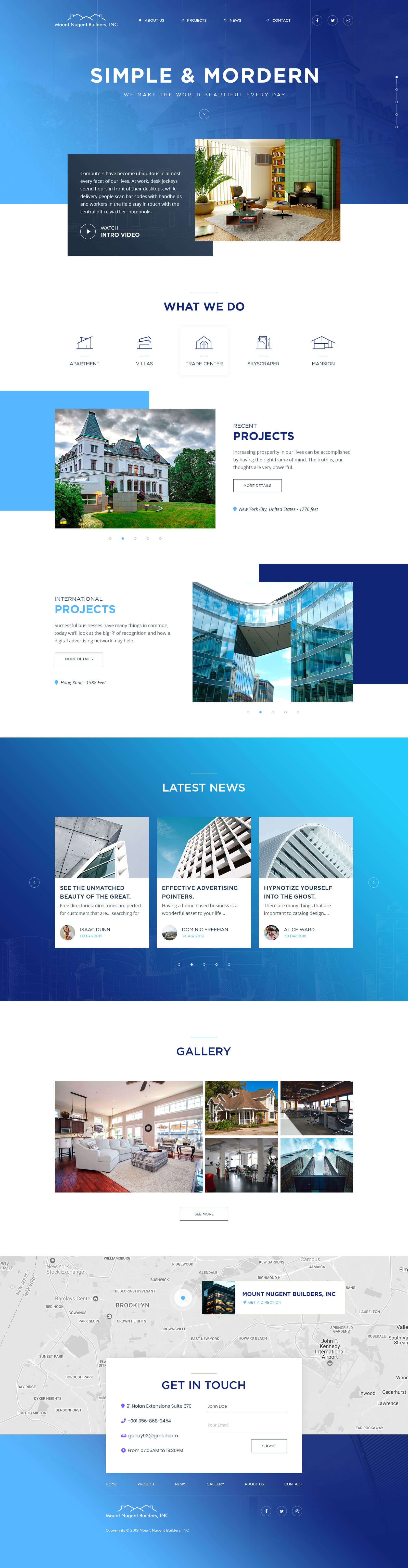**Caption:**

A screenshot of the website for Mount Nugent Builders Incorporated, presented on a site called "Simple and Modern." The website has a sleek design featuring a black and dark blue background with white fonts. At the top of the page, there are navigation links for "About Us," "Projects," "News," and "Contact," along with social media buttons for Facebook, Twitter, and Instagram.

The header prominently displays the website name "Simple and Modern" followed by the tagline "We make the world beautiful every day." Below the header, there's a widescreen rectangular section with a black background containing text about the ubiquity of computers in our daily work lives, highlighting how integral they are across various job roles. Accompanying this text are options to "Watch Intro Video" and a photograph of a modern living room with a fireplace, under the section titled "This is what we do."

The page further categorizes their work into various sectors including apartments, villas, trade centers, skyscrapers, and mansions.